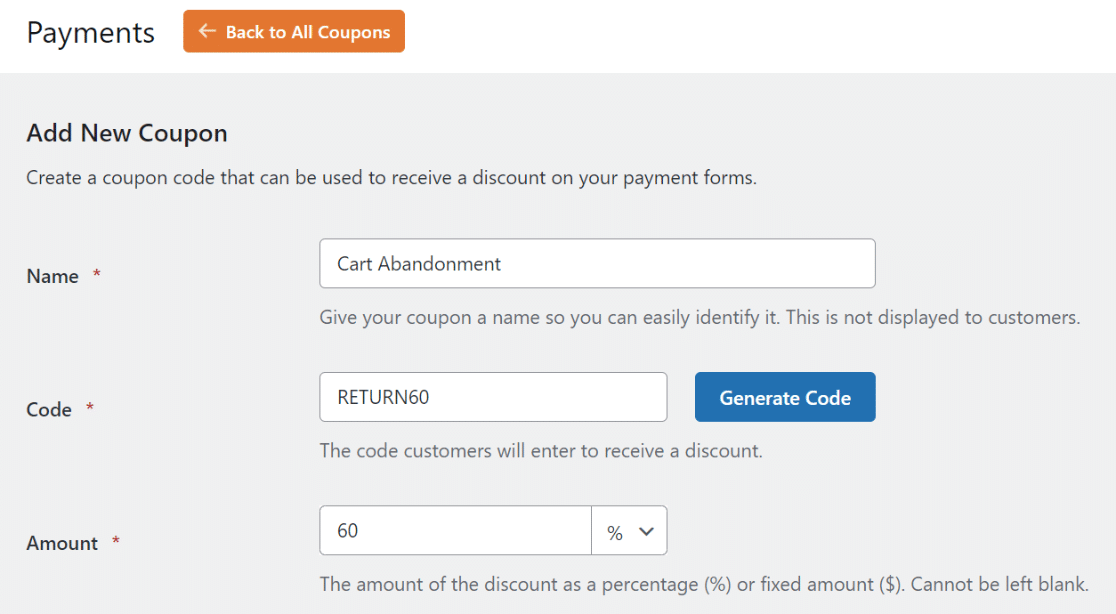**Caption for the Image:**

The image captures the payment section of a website, emphasizing its user interface design. At the top left corner, the word "Payments" is prominently displayed in black on a white background. Adjacent to this, there is a light orange, rectangular button featuring a white, left-pointing arrow, with the text "Back to All Coupons" in white.

Below this, a light gray section is present with the text "Add New Coupon." This is followed by the instruction "Create a coupon code that can be used to receive a discount on your payment forms." 

The section is divided into three parts: 

1. **Name**: Contains a text field labeled "Cart Abandonment," with a note below stating "Give your coupon a name so you can easily identify this. This is not displayed to customers."
2. **Code**: Includes the text "Return 60," with a blue button labeled "Generate Code." Beneath this, it explains, "The code customers will enter to receive a discount."
3. **Amount**: Features a text field with the number "60" and a drop-down menu with a percentage symbol. Below, it clarifies, "The amount of the discount as a percentage or fixed amount cannot be left blank."